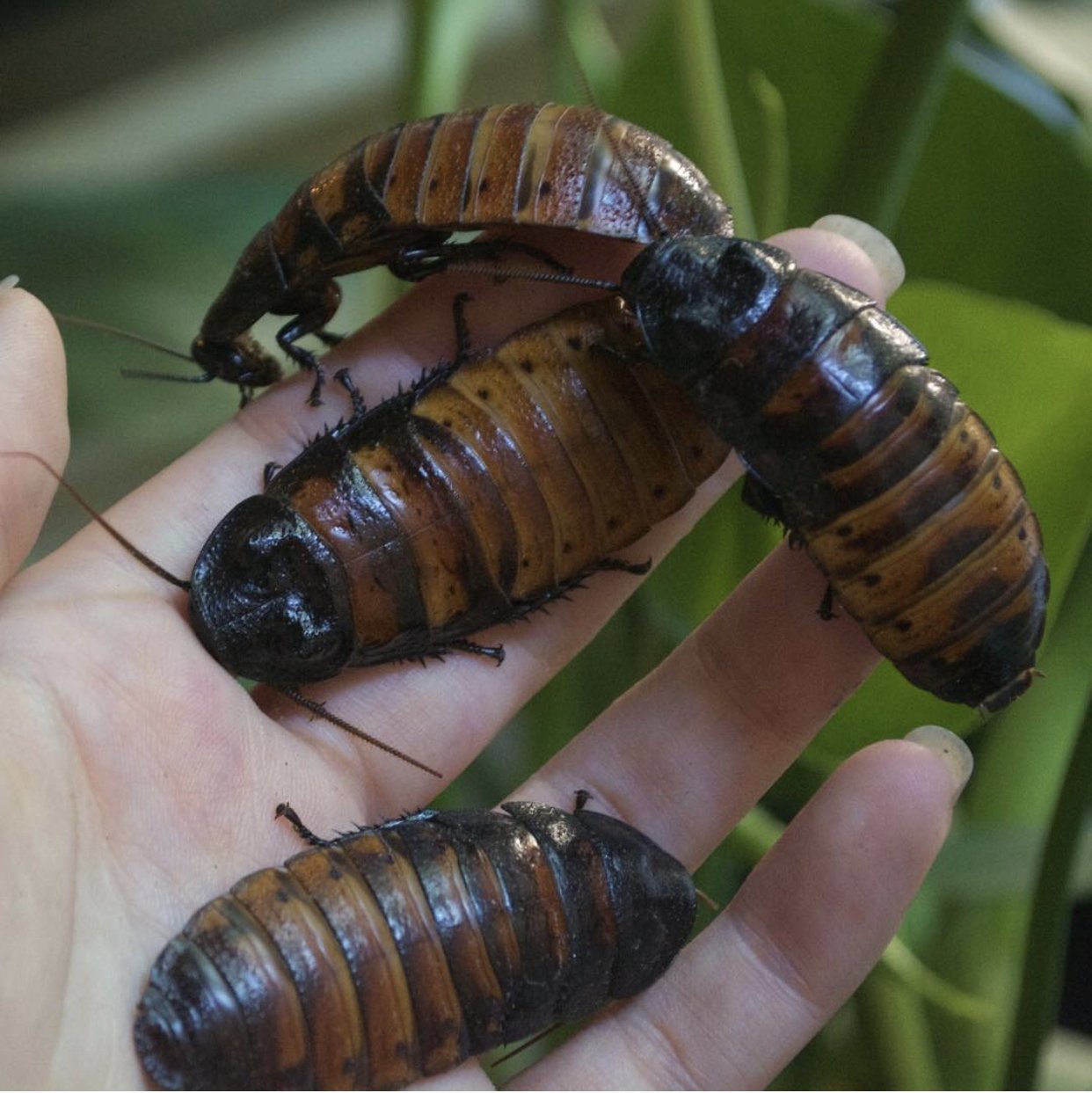The photograph showcases a person's hand emerging from the lower left corner, holding four large, striped black and brown beetles. The hand, adorned with long fingernails, is positioned with the thumb barely visible at the upper left, while the fingers extend upward and to the right. The bottom left hosts a beetle nestled partly in the palm, with its head pointing up and situated between the pinky and ring finger. Above this beetle, on the middle and forefinger, there is an upside-down beetle with its head near the palm and end of the body near the fingertips. Another beetle crawls to the left on the same fingers, with its head on the left side of the finger and its back toward the tip. Slightly below and to the right of this beetle is the fourth beetle, oriented with its head up and to the left and the back end of the body going down and to the right. In the blurred background, hues of green, blue, and white suggest a natural setting with plants. The beetles exhibit a coruscated carapace and have distinctive black antennae and legs.